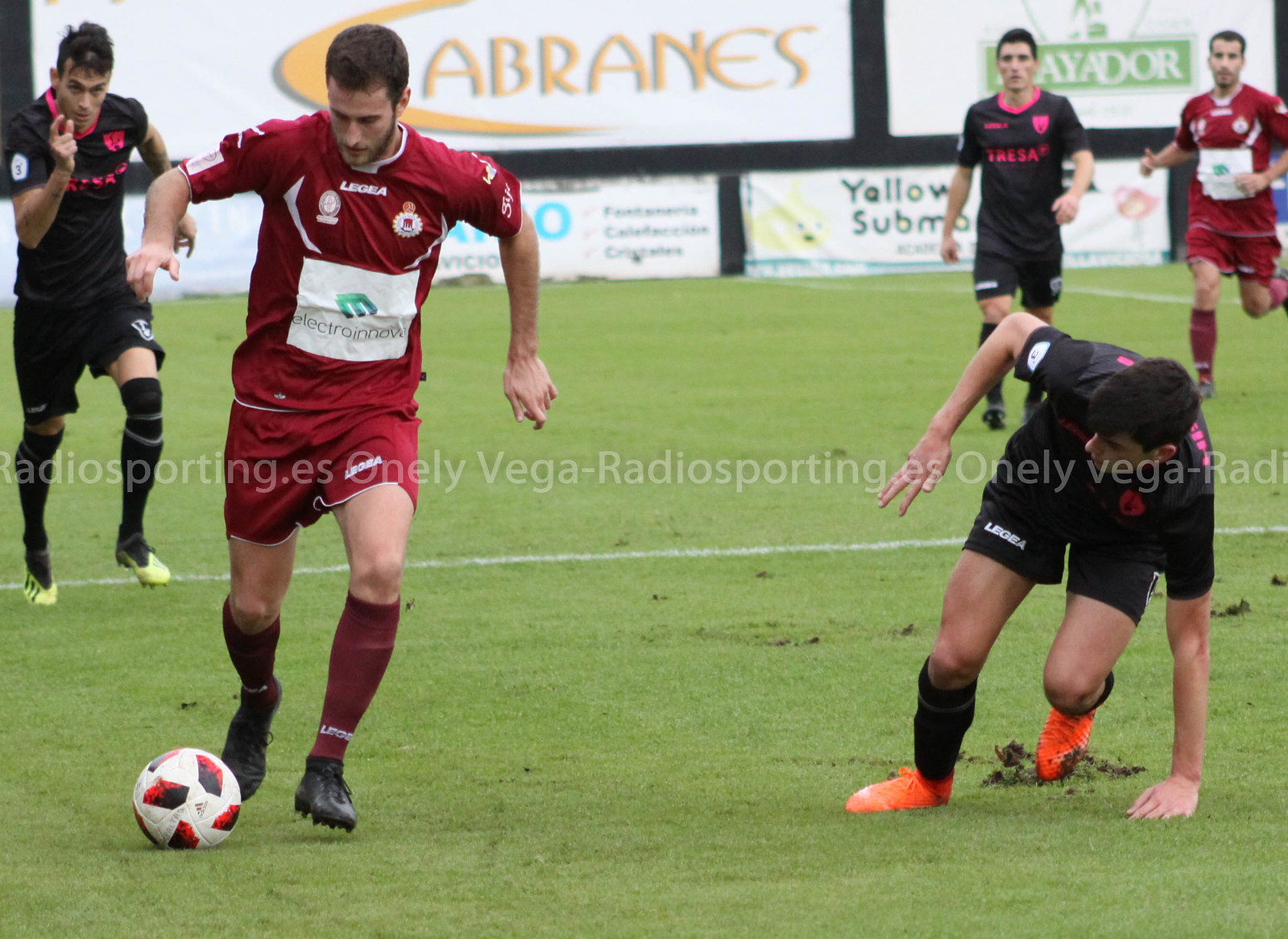In this dynamic soccer match photo, five players are captured mid-action on a lush green field. Three players are from a team dressed in black with pink accents, while the other two players sport red and white uniforms. The focal point is the player on the left in red, who is poised to kick a white soccer ball adorned with black and red designs. Behind him, a player in black and pink is sprinting with intense focus. To their right, another player in black has slipped and is in the process of regaining his balance, with his left hand bracing against the ground and turf visibly kicked up beneath his foot, suggesting possibly slippery conditions. Further to the right, two additional players—one in black and one in red—are seen jogging and observing the unfolding action. The background is filled with various advertisements, including noticeable ones like "Cabranes" and "yellow subma," as well as a middle banner with the repeated inscription "Vega Radio sporting dot ES." This banner runs horizontally across the image, adding to the lively atmosphere of the match.